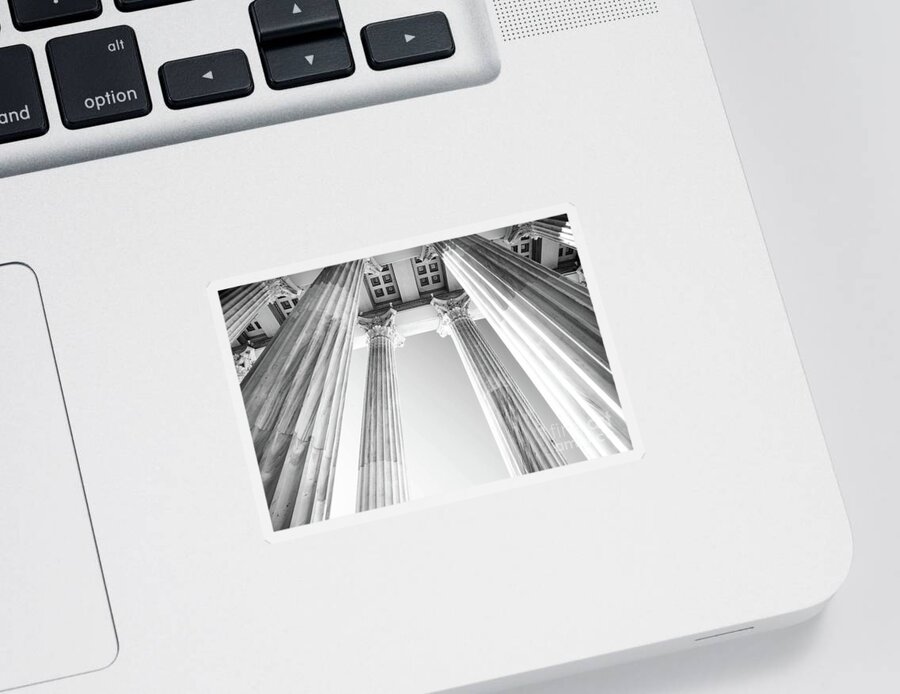The image depicts the bottom right-hand corner of a white Apple laptop against a light gray surface. The laptop features black keys and a prominent trackpad in the bottom left corner of the visible area. Additionally, a short rectangular image, possibly a sticker or a small LCD screen, is situated near the bottom right corner of the laptop, displaying an architectural scene with columns of varying thicknesses ascending towards a ceiling. The keyboard reveals buttons labeled "command" and "option," and near the top can be seen small holes, likely indicating the presence of a speaker. The focus remains on this intricate corner of the laptop with its distinctive components and the mysterious image with the columns.